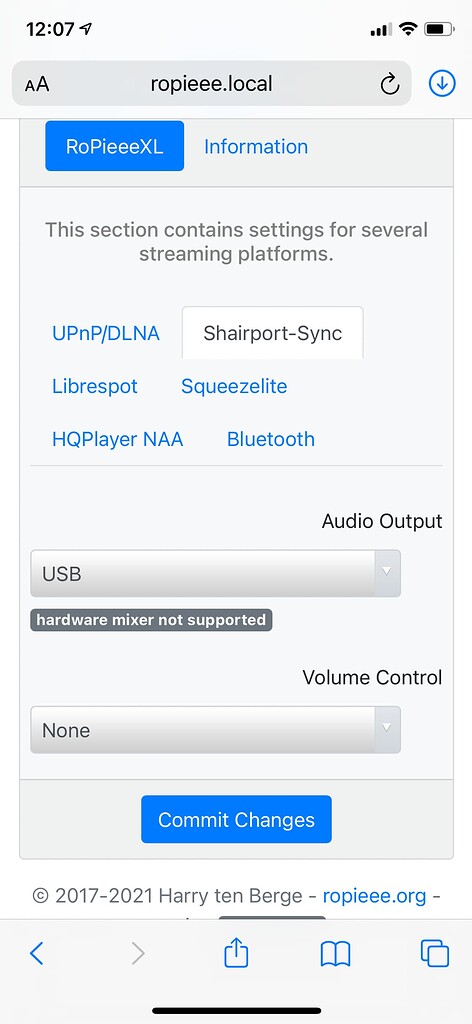The screenshot captures the interface of a website, providing a clear view of various settings and options. At the top of the screenshot, the current time is displayed as 12:07, accompanied by icons on the right side indicating data connectivity, Wi-Fi signal strength, and battery status. The URL visible in the address bar reads "ropee with three e's dot local".

Below the address bar, the interface features a navigation bar with a blue button labeled "Ropieee XL" on the left side and a blue text link labeled "Information" on the right side. The main section of the page is introduced with the text, "This section contains settings for several streaming platforms."

The left side of the settings section lists various streaming platforms and protocols in a vertical arrangement: 
- UPnP/DLNA 
- SharePort-Sync 
- Librespot 
- Squeezelite 
- Bluetooth 
- HQPlayer 
- NAA

On the right side, there are additional settings categories, specifically relating to audio configurations. Under the "Audio Output" heading, the chosen option is marked as "USB." Similarly, under "Volume Control," the selection is marked as "None."

Finally, at the bottom of the settings section, there is a prominent blue button labeled "Commit Changes," presumably allowing the user to apply any adjustments made in the settings.

Overall, the screenshot provides a comprehensive view of the website's user interface, detailing both streaming and audio output settings available to the user.